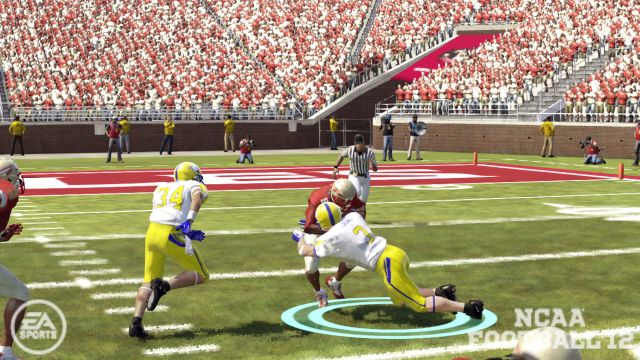This image, captured from the video game NCAA Football 12, showcases a vibrant and intense moment on the football field. The scene depicts two teams in the midst of gameplay, with players dressed in yellow uniforms competing against those in red uniforms. In the background, an enthusiastic crowd fills the stadium, adding to the electrifying atmosphere. A referee, clad in black and white stripes, is visible overseeing the action. A watermark reading "EA Sports" is positioned at the bottom left corner, while the game title, "NCAA Football 12," is prominently displayed at the bottom right. The detailed graphics and dynamic scene encapsulate the excitement and realism of college football in this iconic video game.